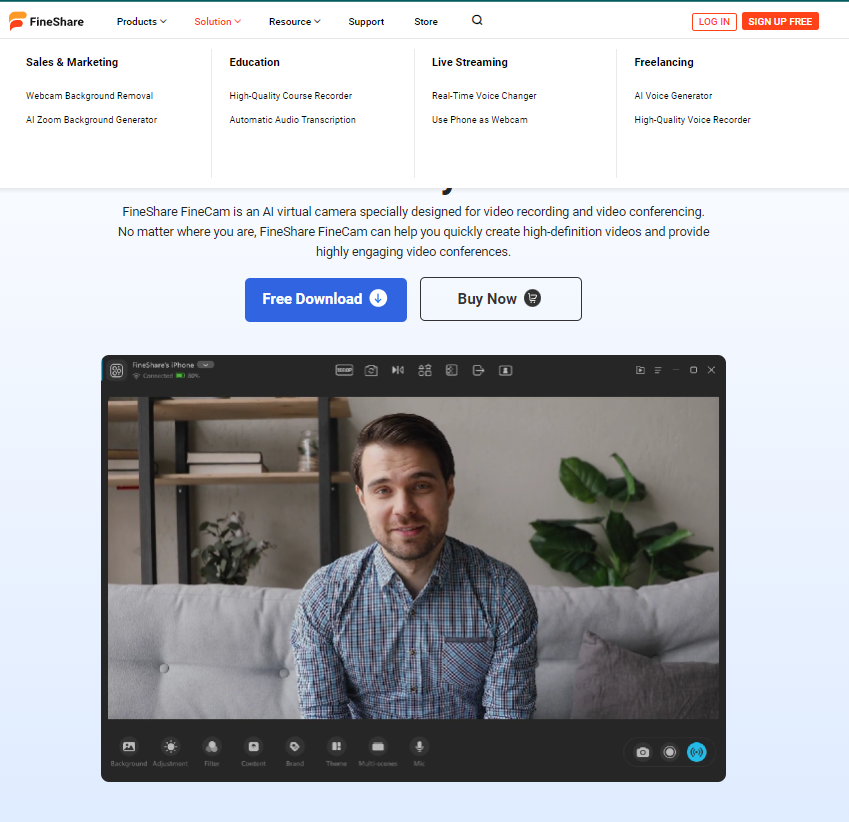This image is a portrait-oriented screenshot of an application interface featuring a thin bluish-green border running across the top. Below this, a thin gray border separates the green border from some text in black font that reads "Find Shirts", accompanied by a logo with an orange top and a red base. 

The navigation menu situated at the top includes several options: "Products" with a dropdown menu, "Solution" highlighted in red with a dropdown menu, "Resource", "Support", "Store", and a magnifying glass icon for search functionality. Adjacent to this menu, there are two distinct red buttons: one with red font that says "Log In" and another with white font that says "Sign Up Free". 

Below these buttons, the interface is divided into vertical subcategories with their respective options: "Sales and Marketing", "Education", "Live Streaming", and "Freelancing". A brief block of text follows these categories. 

Further down, there are two rectangular buttons: a blue one with white text that says "Free Download" featuring a downward-pointing arrow inside a circle, and a gray-bordered "Buy Now" button with gray font next to a shopping cart icon. Lastly, at the bottom of the screen, there is a gray rectangular section that contains an image of a man who appears to be speaking directly to the viewer.